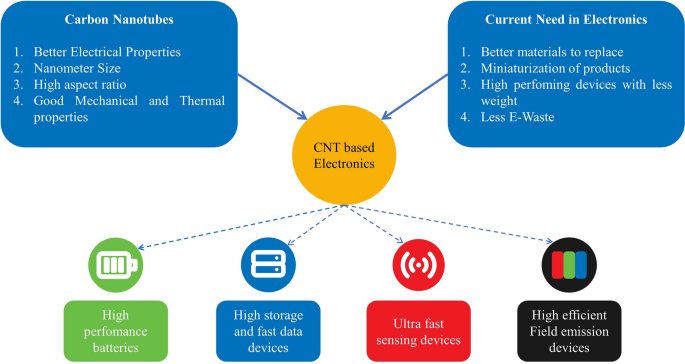The illustration is a detailed flowchart set against a white background, featuring two blue rectangles with rounded corners, a central yellow circle, and multiple arrows and icons.

In the upper left corner, there's a blue rectangle labeled "Carbon Nanotubes" in white text, listing four key attributes: 1) better electrical properties, 2) nanometer size, 3) high aspect ratio, and 4) good mechanical and thermal properties. An arrow from this rectangle points toward the central yellow circle labeled "CNT-Based Electronics."

In the upper right corner, another blue rectangle labeled "Current Need in Electronics" in white text lists four critical requirements: 1) better materials to replace, 2) miniaturization of products, 3) high-performing devices with less weight, and 4) less e-waste. An arrow from this rectangle also points toward the central "CNT-Based Electronics" circle.

Four dashed blue arrows emanate from the central yellow circle, indicating different applications. The arrow to the far left, colored green, points to the label "High-Performance Batteries" and is accompanied by a circular icon depicting a battery. The next arrow labels "High Storage and Fast Data Devices," associated with a blue circular hardware icon. The third arrow, leading to the label "Ultrafine Sensing Devices," is paired with a red circle illustrating a Wi-Fi signal. The far-right arrow labels "High-Efficient Field Emission Devices" and is marked by a black circle containing three vertical bands colored red, green, and blue.

Overall, the diagram effectively highlights the potential of CNT-based electronics to meet current needs in electronics through various high-performance applications.